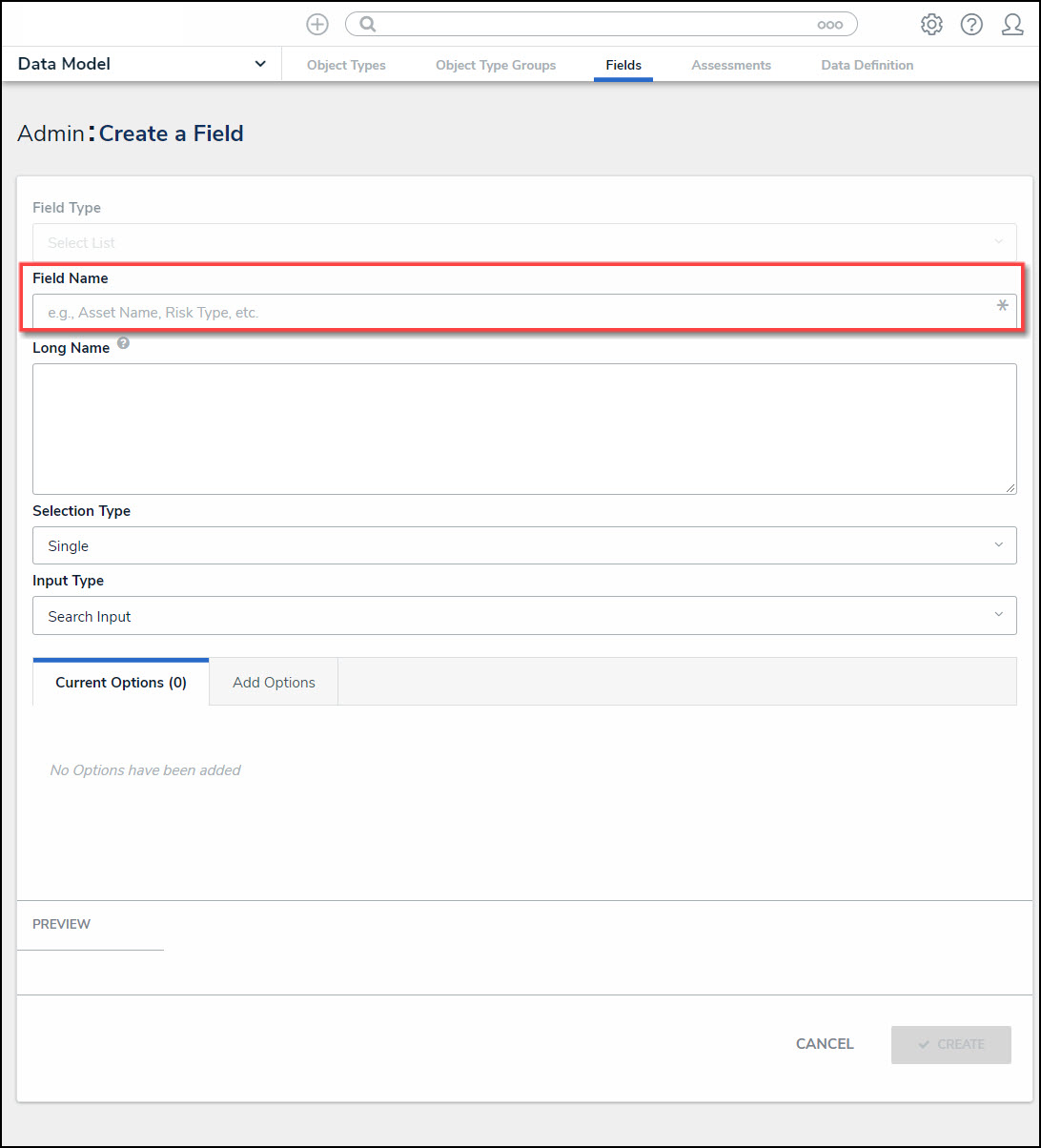**Caption:**

This color image in portrait orientation appears to be a screenshot taken from either a phone or computer. It displays a software interface, specifically a settings window for configuring a data model. The window has a very functional, no-frills design and contains no imagery, focusing solely on the practical aspects of data entry. 

At the top left corner, the title "Data Model" is prominently displayed, with several tabs to the right offering different options: Object Types, Object Type Groups, Fields, Assessments, and Data Definition. In this screenshot, the user has selected the "Fields" tab. 

The interface presents a form to be filled out, with various sections and options. The current view shows settings under "Admin: Create a Field." Here, the user can choose the field type, field name, and other parameters, although no field type has been selected yet. The field name section is notably emphasized with a red rectangle, drawing attention to it as a crucial part of the form.

Further down, the form includes additional sections for "Long Name," which allows for a more extended text input, "Selection Type," "Input Type," and "Current Options," though these sections are not filled in. The overall presentation suggests the user is in the process of setting up or editing a field within the software, highlighting the field name as an important focus.